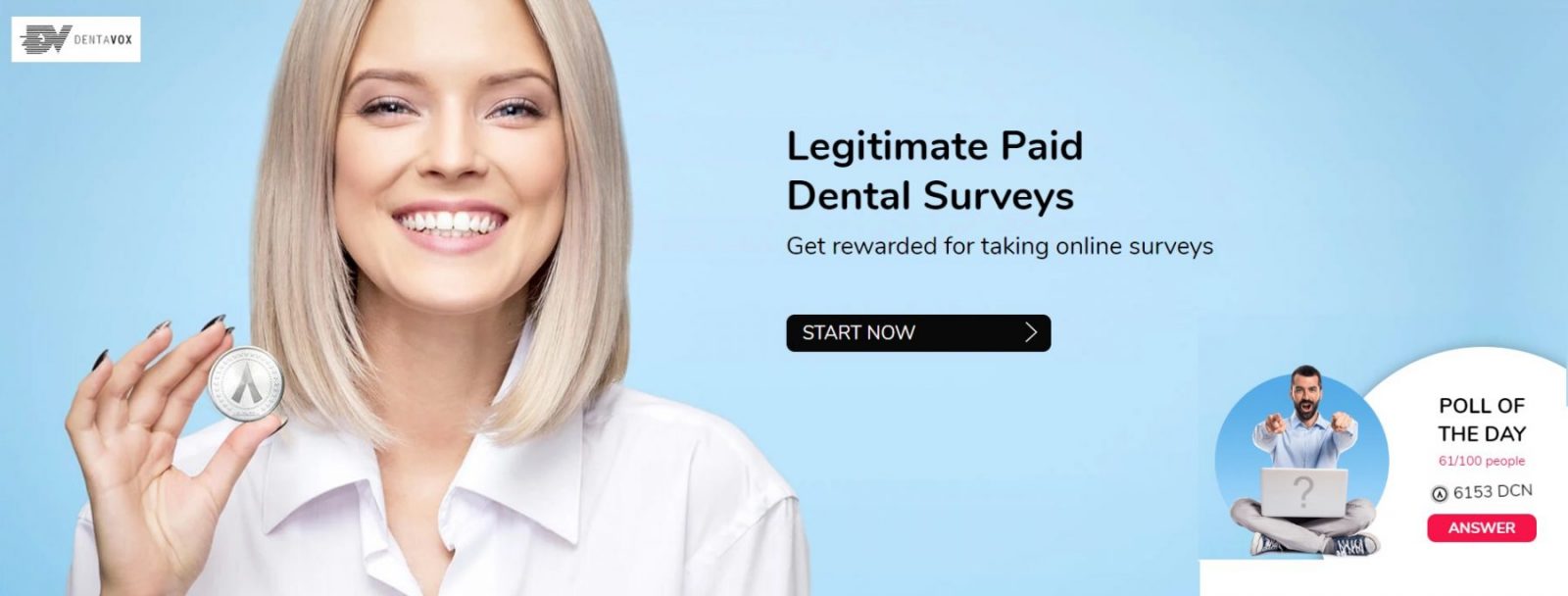The image features a light blue background with a prominent section showcasing a woman with blue eyes and a cheerful smile, revealing her teeth. She is wearing a white collared shirt and holding a coin. Her backdrop includes the logo "DV" next to the text, "Legitimate Paid Dental Surveys - Get rewarded for taking online surveys." 

Below this, there is a black rectangle with the text "Start Now" in white.

Adjacent to the woman’s section, a man is depicted sitting cross-legged ("Indian style") with a laptop resting on his lap. He is dressed in a light blue collared shirt, gray pants, and gray sneakers. His arms are extended with both hands pointing towards the camera. The backdrop near the man features the text, "Poll of the Day: 61 out of 100 people" in red. Below this, there is a red rectangle with the word "Answer" in white.